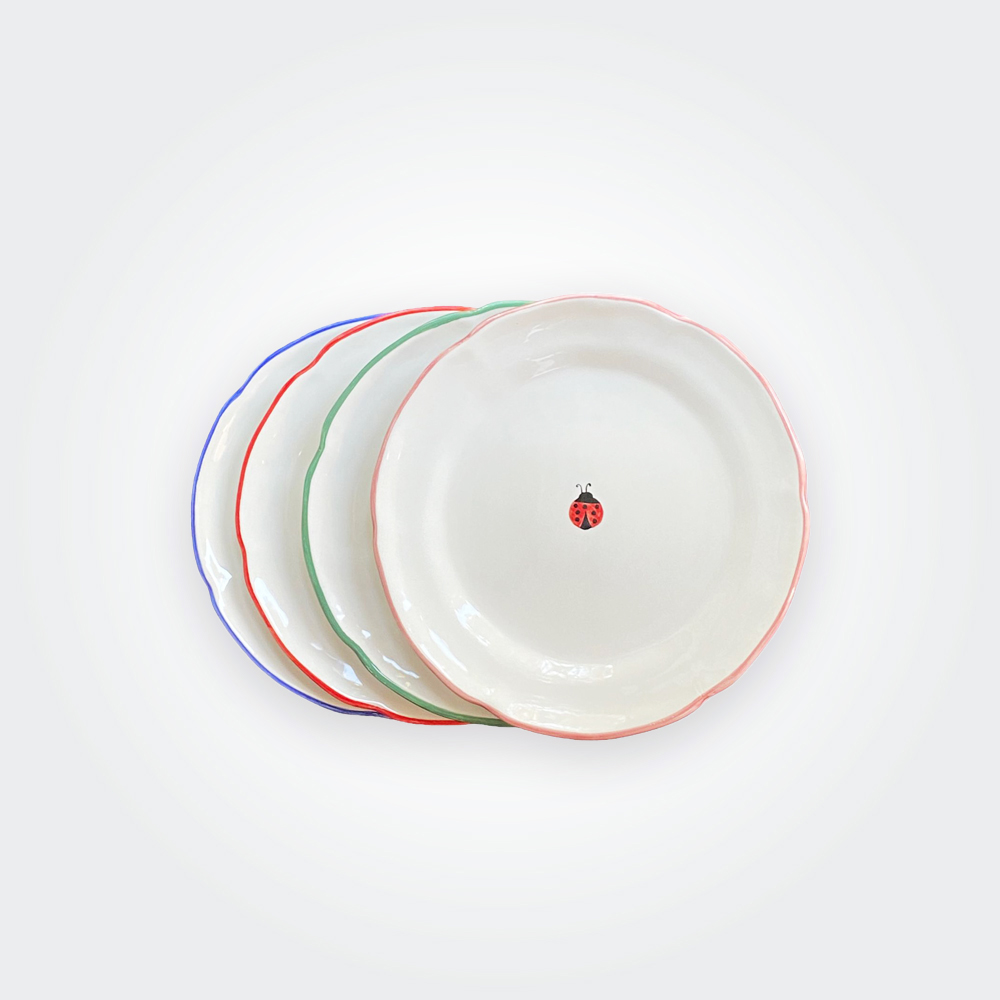This image features a series of four fragile, white glass dinner plates, stacked and slightly offset like a fanned deck of cards, allowing glimpses of each plate’s rim. They are arranged on a very light gray background, shaded darker on the upper left. The top plate is adorned with a delicate illustration of a ladybug in the center, showcasing a black head, red wings with black dots, and small black antennae. The rims of the plates, each finely edged in different colors, add a touch of elegance. The top plate has a light red or pale orangey-red border, the second plate is edged in green, the third in a dark red, and the fourth in blue.